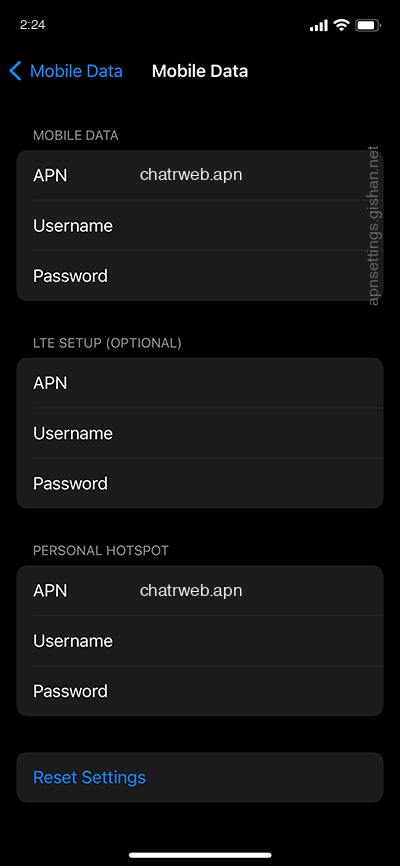This image captures a smartphone screen displaying mobile network settings. The screenshot, taken from a cellphone, features a black background. At the top left corner, the time reads 6:42. Adjacent to the time, a blue arrow points left, followed by the label "mobile data" in blue text. About an inch to the right, "mobile data" is repeated in white text. Further right, the battery icon is nearly full.

Below this, various network settings are shown: 

1. **APN**: "CHATWEB.APN"
2. **Username**: Empty Field
3. **Password**: Empty Field
4. **LTE Setup (Optional)**:
   - APN: Empty Field
   - Username: Empty Field
   - Password: Empty Field

In light gray text, the label "Personal Hotspot" is visible, followed by:

1. **APN**: "chatrweb.apn"
2. **Username**: Empty Field
3. **Password**: Empty Field

Further below, a blue rectangular button labeled "Reset Settings" is displayed. This marks the end of the informational text on the screen.